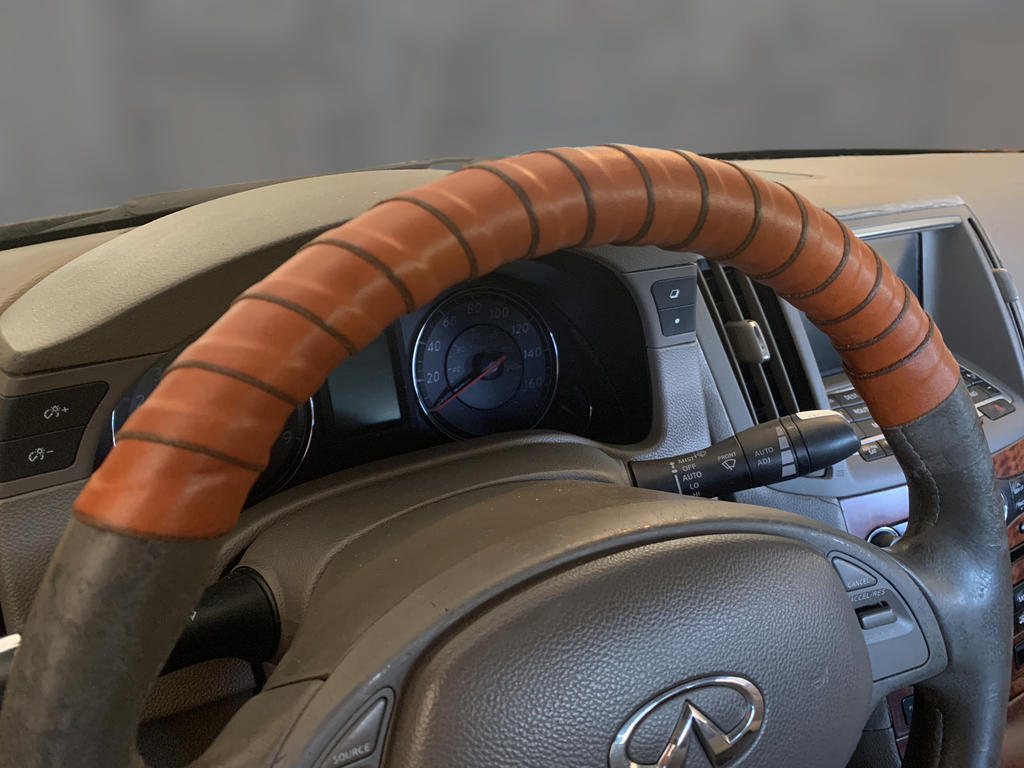This photograph showcases the interior of an older vehicle, likely from the mid-2000s, focusing prominently on the steering wheel. The steering wheel, which dominates the image, is primarily gray with the top half featuring brown sections that resemble the texture and color of a football. This brown portion appears to be made from a different material. Centrally placed on the steering wheel is a symbol similar to that of Nissan's Infiniti. 

Behind the steering wheel, a speedometer reaching up to 160 miles per hour is visible. On the right side of the wheel are the windshield wiper controls, as well as a radio system and a possible video navigation system. The dashboard around these elements has a faux wood finish, adding to the slightly aged aesthetic of the interior. The photograph likely has the windshield edited out or obscured by a gray and white fog effect, suggesting the car might be covered or stored. Overall, the car exhibits wear, indicating it is not a new model, but instead has been used for several years.